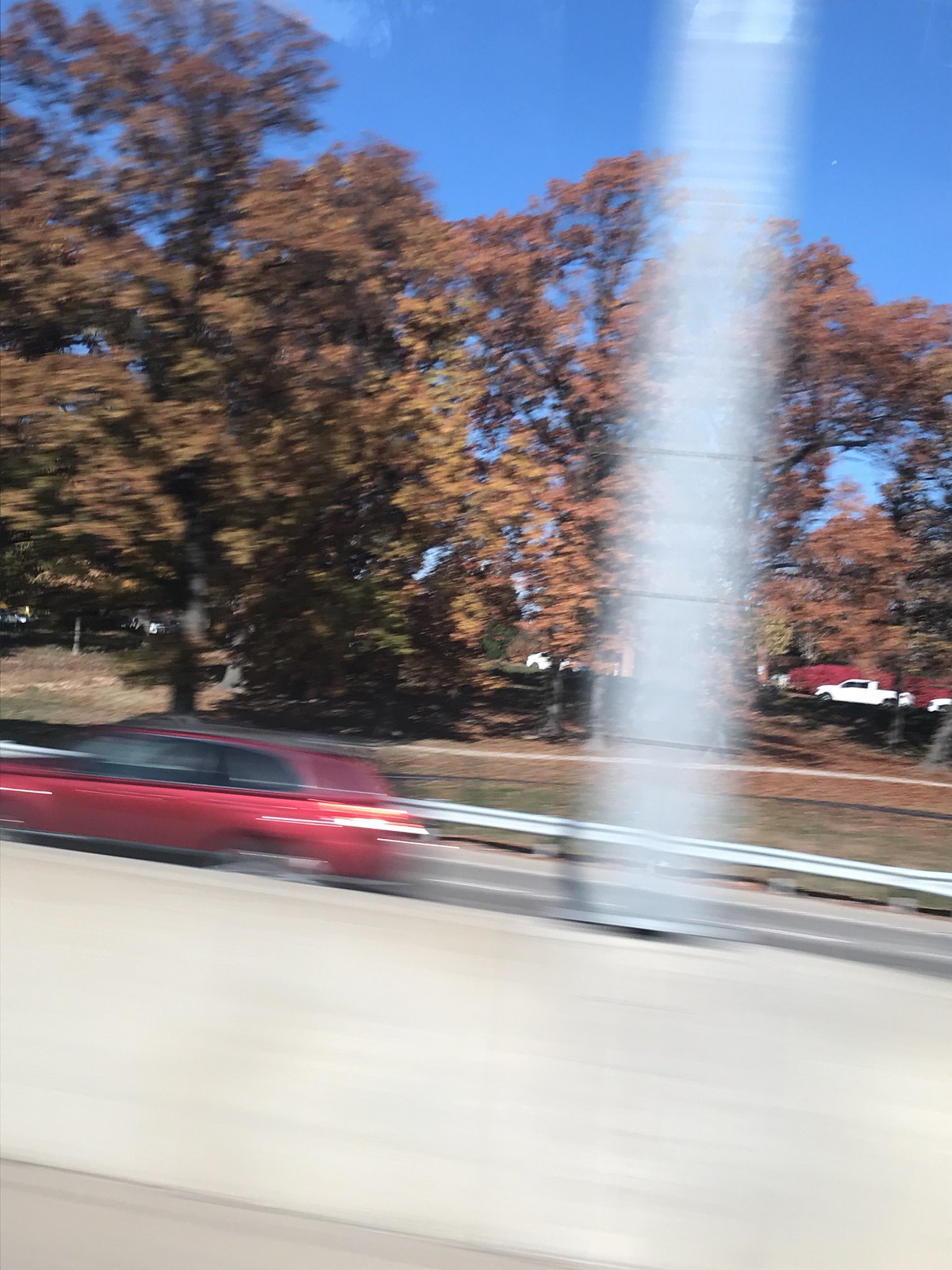In this color photograph taken during the daytime, we're positioned on one side of a freeway, possibly within a moving vehicle that is heading right. The shot captures the view through the side window, beyond the central barrier of the freeway. On the opposite side of the barrier, a red car is seen traveling in the left direction. Behind this scene, there is a hillside adorned with tall trees displaying vibrant fall foliage. Further beyond the trees, a parking area is visible, featuring a white truck and a small white car. The image is characterized by its blurriness and noticeable glare, which appears to originate from the right side of the frame, likely the result of sunlight reflecting off the vehicle window.